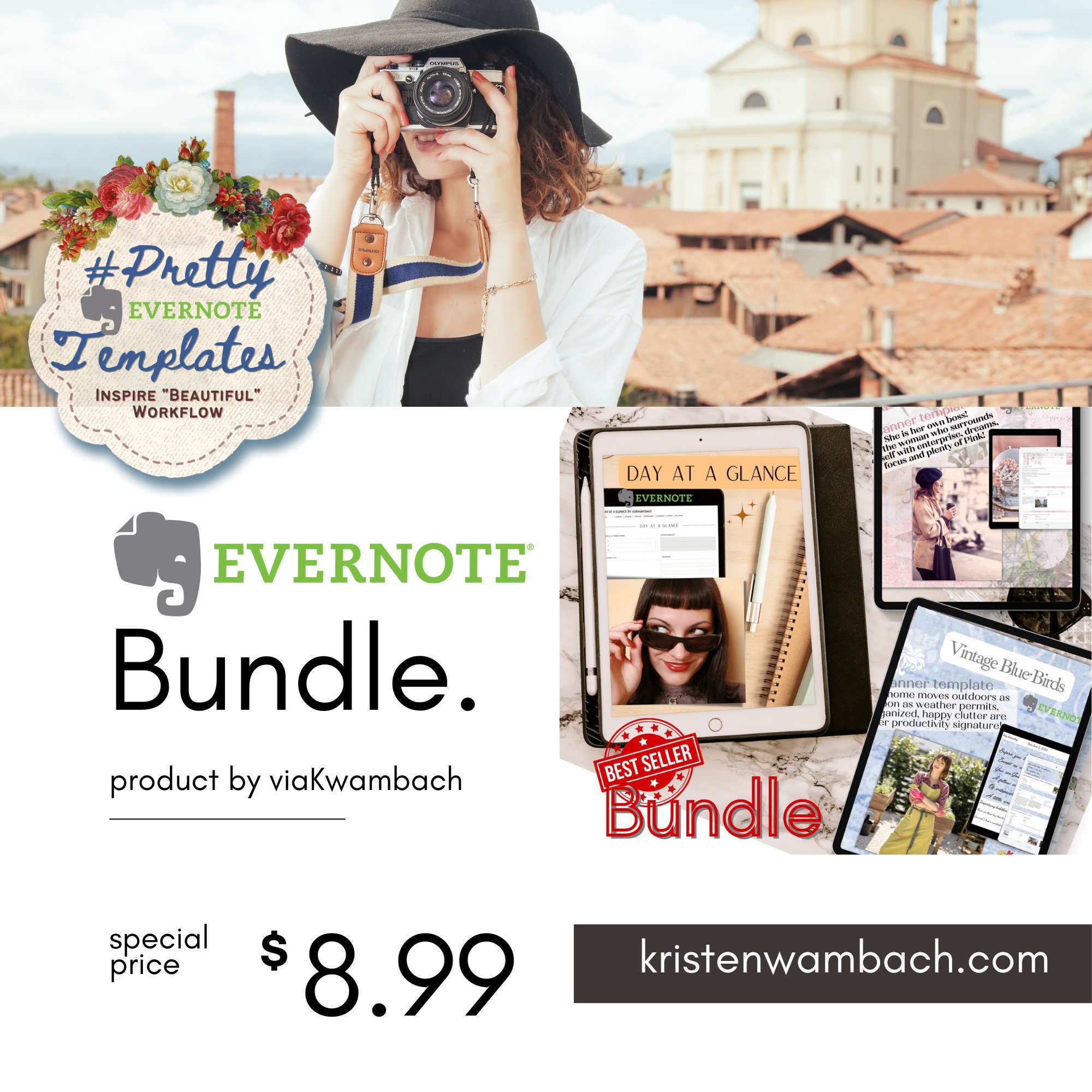The image is an advertisement for the Evernote Bundle, available at KristenQuambach.com for a special price of $8.99. At the top of the ad, a woman wearing a black sun hat, a white cardigan, and a black shirt is seen taking a photo, set against the backdrop of a European cityscape. The city features old buildings with orange roofs, a tall building that stands out, and a church with an orange roof. To her left in the background, there's a chimney emitting smoke under a blue, cloudy sky. A floral embroidery frames the top of the ad.

The central text highlights "Hashtag PrettyEvernoteTemplates," promising to "Inspire Beautiful Workflow." The advertisement features the iconic Evernote elephant logo turned to the side, with "Evernote" written in bold green. Below, "Evernote Bundle Product by Via Quambach" is written in black with a line underneath. 

To the right, there are three tablet screenshots displaying various day planners titled "Day at a Glance." A round circle within a bar declares the product a "Best Seller Bundle." Lastly, a black box with white lettering directs potential customers to visit KristenQuambach.com.